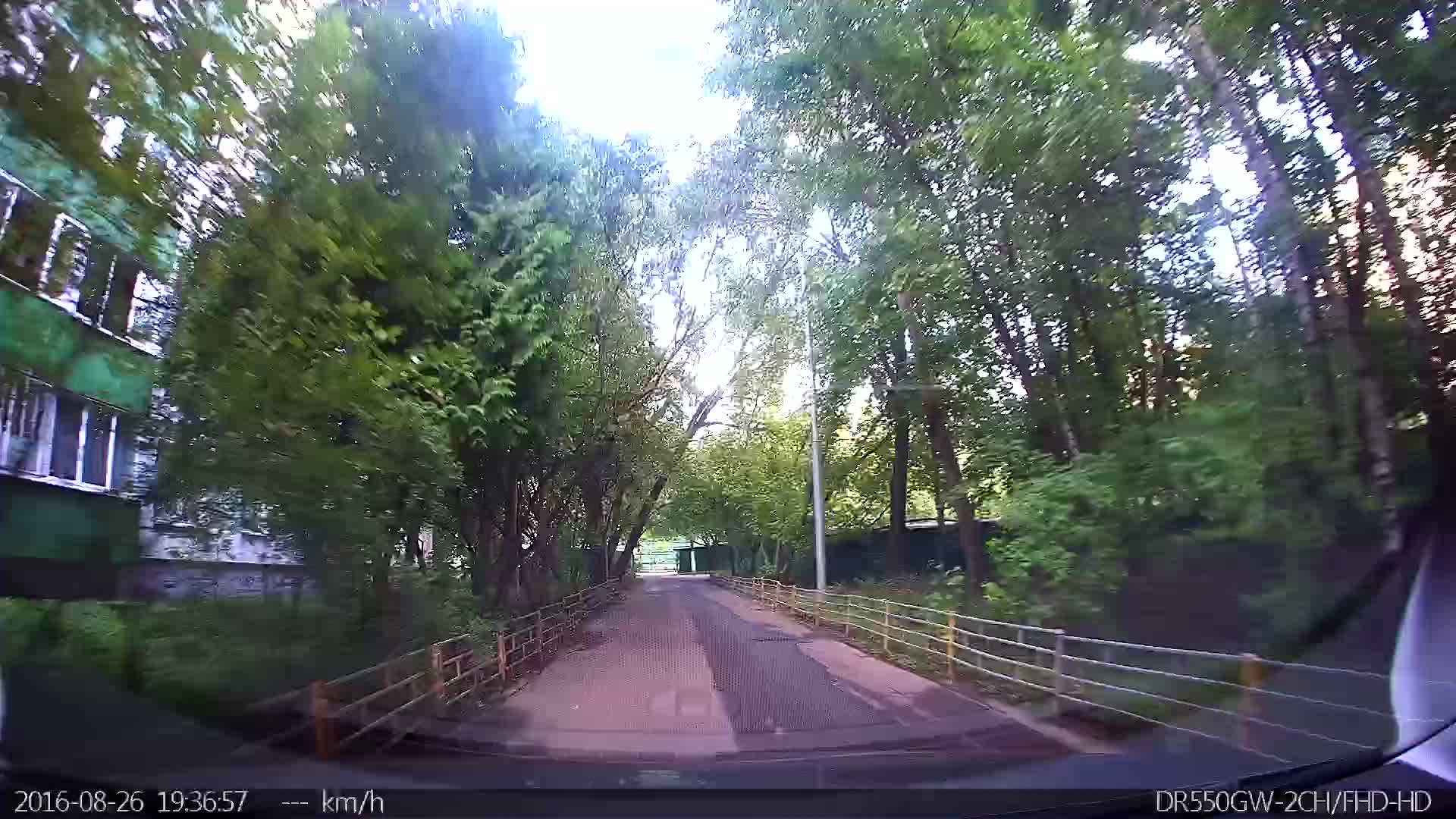This image is a dash cam photograph taken outside along a path that resembles a narrow road. The path is clay-colored and lined with wooden, four-line guardrails on both sides, which are there to offer minimal protection. Tall brown trees with green leaves line both sides of this path, and sunlight filters through their branches. To the left, there's a tall building with green awnings stacked up along its side, and the windows are framed in white. The patch of green grass at the bottom of the building is complemented by the sunlight. A long, silver light post is visible in the background of the photograph, indicating that it is daytime as the light is not on.

The photograph also includes text at the bottom edges, with the left side displaying the date "2016-08-26" and the time "1936:57". The text also includes "KM/H", but the speed is blank. On the bottom right, further text reads "DR550GW-2CH-FHD-HD". The slightly curved effect might be an intentional feature or a result of being viewed through the dash cam, suggesting a subtle fish-eye lens distortion. The path does not appear to be a main street, more like a back alley bordering the trees and the building. This detailed composition provides a meticulous snapshot of a serene, suburban moment captured in time.